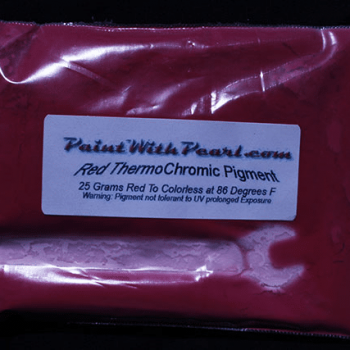This image depicts a vacuum-sealed plastic bag set against a black background. The bag, largely red with a transparent front panel, reveals a wrench inside. Prominently displayed on the bag is a white label with black text reading "paintwithpearl.com." The primary description on the label identifies the contents as "red thermochromic pigment" in 25-gram quantities. Additional details specify that the pigment changes from red to colorless at 86 degrees Fahrenheit and warn that it is not tolerant to prolonged UV exposure. The image is zoomed in, occupying the entire frame, and appears to have a commercial context, likely designed for direct sale on the website mentioned.